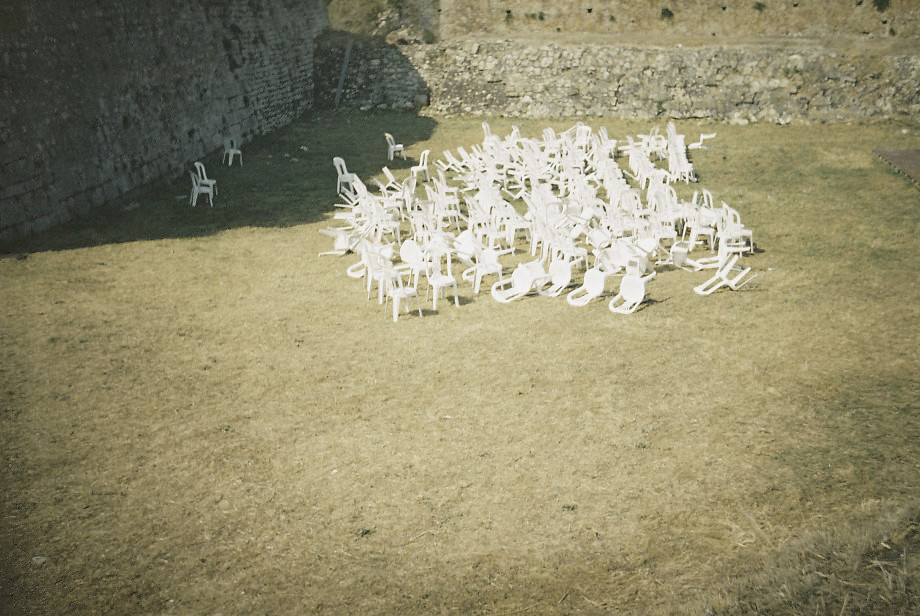In the image, a chaotic cluster of white plastic lawn chairs is strewn across a field of dead grass, creating a poignant scene of disarray. The majority of the chairs are haphazardly placed in the center, with some tipped over and others standing upright. A few chairs are scattered closer to the old, crumbling stone walls that frame the background and sides of the field. The sunlight indicates that it’s daytime, and a large shadow cast by a wall is visible in the top left corner, adding to the sense of neglect and abandonment. The perspective of the photo, taken from a slightly elevated vantage point, gives an almost aerial view of the scene, which adds to the impression that the area is either very small or the chairs are miniature. The overall atmosphere suggests a once-organized space now in disarray, possibly due to natural elements like wind.